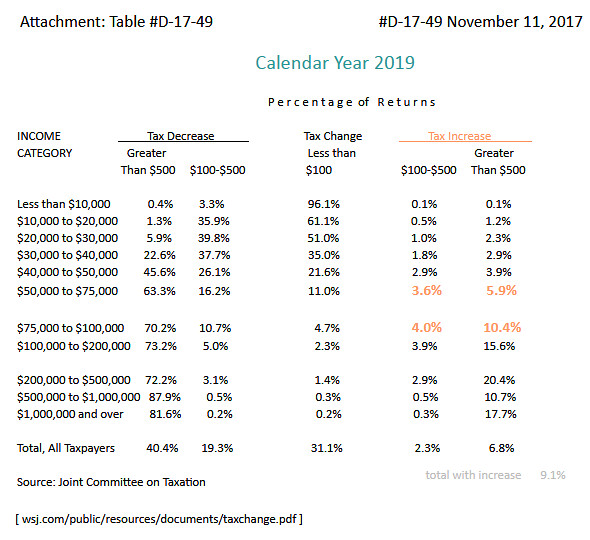The screenshot displays a detailed table predominantly in black text on a white background, meticulously organized to convey tax return data. In the top left corner, it reads "Attachment Table Number D1749," and mirrored in the top right is "Number D1749, November 11th, 2017." Centered below, green text announces "Calendar Year 2019." Following this, black text labels the table as "Percentage of Returns." The table is divided into columns with headings: "Income," "Tax Decrease," "Tax Change," and "Tax Increase," each accompanied by rows detailing various dollar ranges. Some percentages in the "Tax Increase" column are highlighted in peach. The bottom of the table credits the source: "Joint Committee on Taxation," and lists a URL within brackets, directing to a document at "wsj.com/public/resources/documents/taxchange.pdf," located in the bottom left. This screenshot meticulously charts the tax variations for the specified calendar year across different income levels.